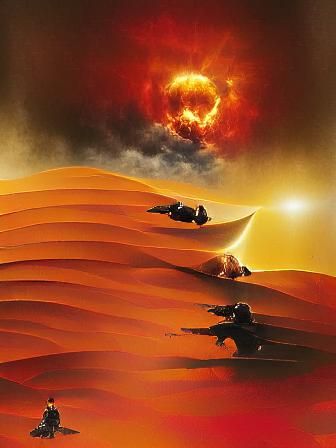This digital artwork depicts a dramatic, futuristic battle scene set against a desolate landscape of orange and red sand dunes that dominate the middle and left side of the image. Central to the scene is a soldier, identifiable by his kneeling posture and futuristic rifle, poised in the sand. Above him, a spaceship hovers at a distance, while a brilliant, yellow sun shines intensely from the middle-right part of the composition. A surreal, perfectly round explosion occupies the top-middle, with a dynamic mix of yellow cracks and surrounding orange hues, emanating black smoke from its base. The sky is tumultuous with shades of dark red, orange, and yellow blending into a smoky, fiery expanse, casting shadows and highlighting the gravity of the scene. Scattered throughout the landscape are shadowy figures and black rocks, enhancing the sense of chaos and tension in this vividly detailed, imaginative artwork.